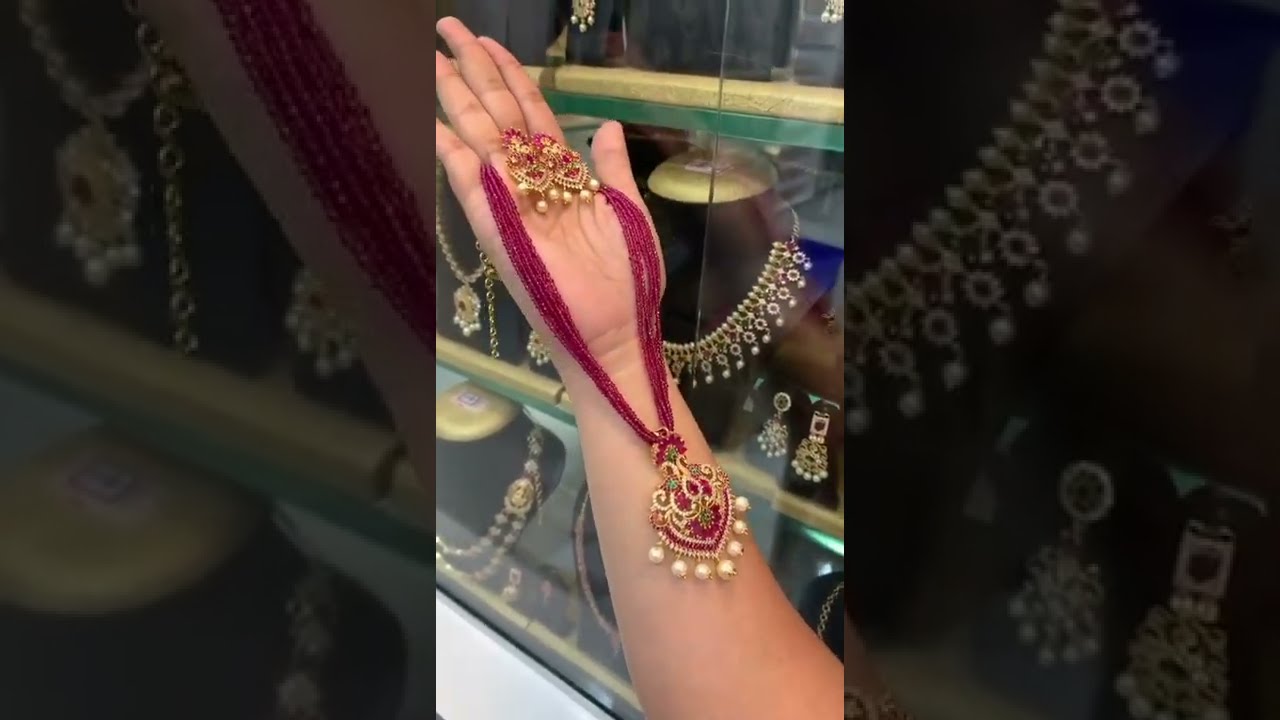This framed artwork features a central, well-illuminated image surrounded by two darker close-up shots, forming a rectangle of three side-by-side pictures. The central image showcases a light-skinned woman's hand, reaching from the bottom right to the top left, holding an elaborately designed necklace. This necklace, potentially Indian or Pakistani in style, features deep magenta yarn with intricate gold adornments and minute green accents. The central pendant is heart-shaped with detailed golden curves and small golden spheres at the bottom. Flanking this main piece, two similar pendants, possibly earrings, are visible.

Behind the hand, a jewelry store setting unfolds, with rows of glass-encased shelves displaying gold-colored necklaces on mannequin necks. The left close-up image highlights another necklace with a bell shape, featuring a hole on the left side and decorative white pearl-like spheres. A partial view of a mannequin is also visible, though it remains unadorned. On the right, another close-up reveals a golden necklace curving towards the mannequin's neck, adorned with a sequence of diamond, flower, and sphere shapes. Two additional golden accessories resembling snowflakes with hanging spheres are also visible in this shot. The scene, likely indoor with fluorescent lighting, encapsulates the elegance and intricate craftsmanship of the jewelry.